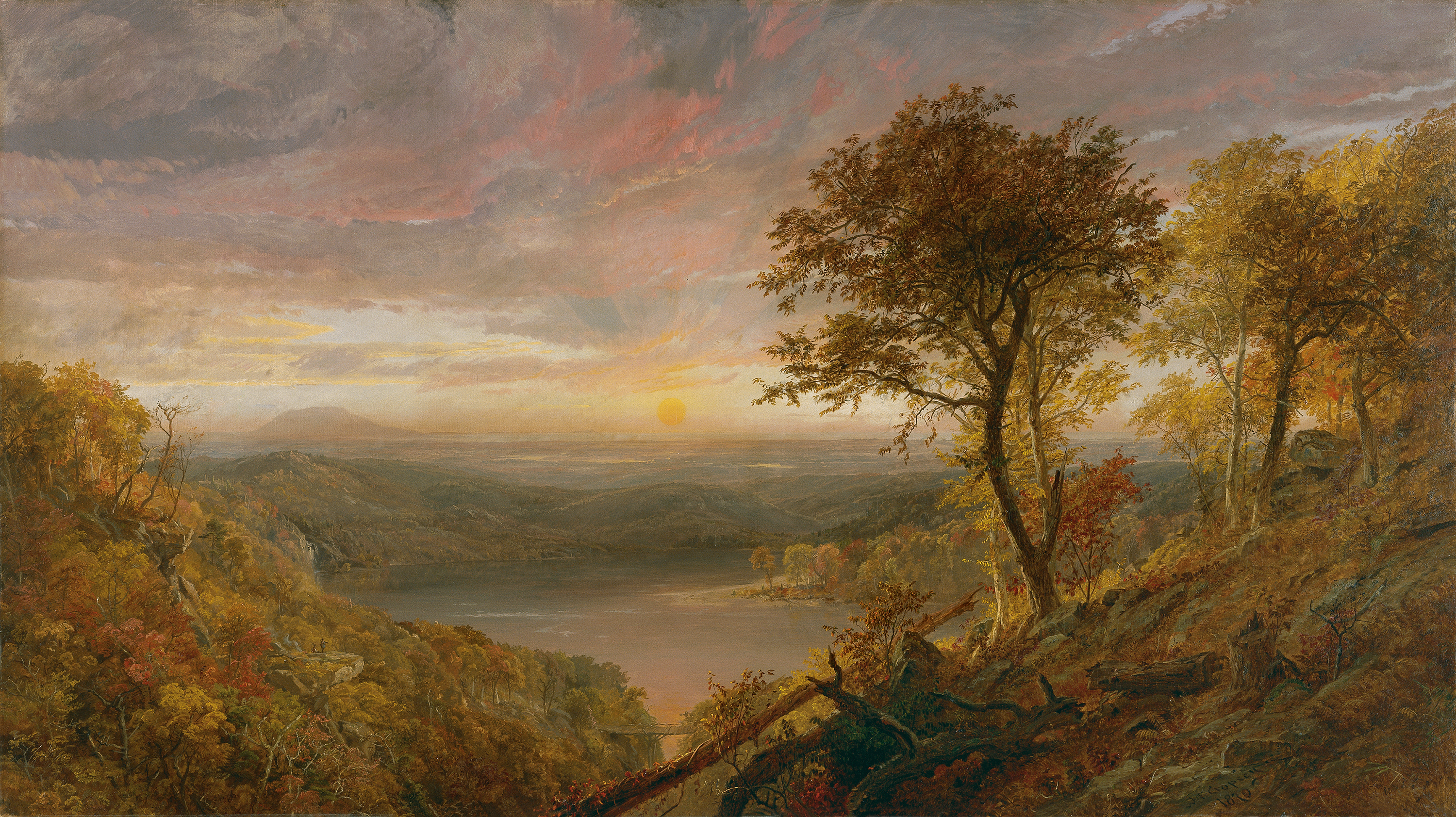This detailed painting captures a serene valley scene during the fall, showcasing a vivid and picturesque landscape. The foreground features a hill rising from the bottom right corner, adorned with trees sporting yellow, orange, and red leaves, indicative of the seasonal transition. To the left, additional brush with similar fall colors reinforces the autumnal theme. The middle ground reveals a wide C-shaped body of water, with its open end facing to the right, leading to a sandy spit topped with trees by the beach. A winding river runs through the lower center of the painting, guiding the viewer's eye towards the water. In the background, rolling hills and a distant mountain frame the horizon, where the sun is either setting or rising, casting a warm yellow glow across the sky. The sky itself is a mesmerizing blend of sunset hues—soft yellows, pinks, oranges, and scattered grays. The entire scene is bathed in the gentle, fading light of dusk or dawn, making for a tranquil and picturesque depiction of nature in watercolor form.